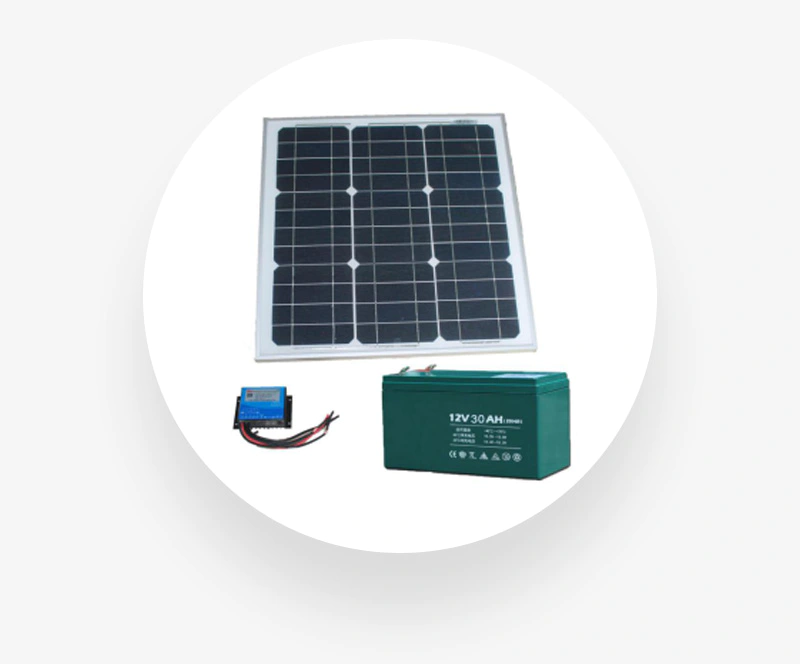This color photograph features a square image with a very light gray background and a large white circle centered in it. Inside the circle, there is a central black and white grid structure that resembles a solar panel or air conditioner filter, bordered by a white frame. The grid pattern within this structure consists of an alternating arrangement of squares and rectangles filled with black.

Positioned at the lower right of the circle is a large, green, rectangular battery pack. The battery pack prominently displays "12V 30AH" along with some smaller, unreadable white text beneath it. On the lower left side of the circle is a small blue box, connected by red and black wires curving outward. The photograph is devoid of any text or border, emphasizing the devices against the minimalistic gray background.